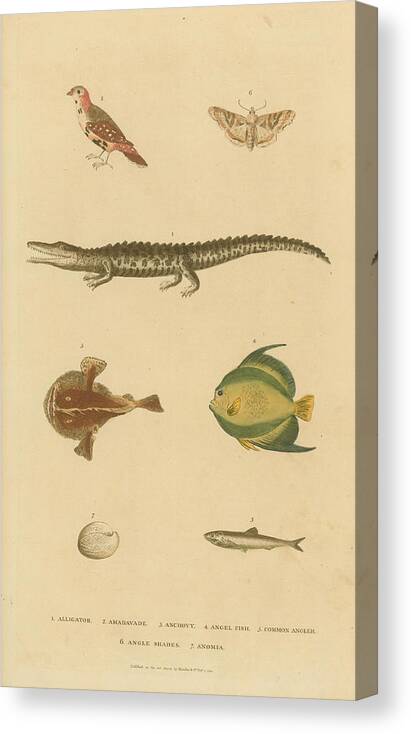This is a product photograph of a canvas print designed to be hung on a wall, showcasing various species of animals and insects. The canvas background is a neutral canvas color. Located at the top left is a small, speckled bird with brown and red plumage. Directly to the right, the canvas features a moth. Beneath these, in the middle section, is an alligator. Below the alligator are two fish: the one on the left is a flat, bottom-dwelling fish with a brown body and eyes positioned atop its head, while the one on the right is a green fish with a crescent-moon shape and long fins on the top and bottom, appearing somewhat angry. On the bottom row, the left image depicts a small, unidentifiable circular object. To the right of it, there is a small, silver fish resembling a minnow or sardine, characterized by very pointed back fins. The bottom of the canvas contains text that identifies each drawing with numbers and names; however, only the word "Alligator" is clearly readable.